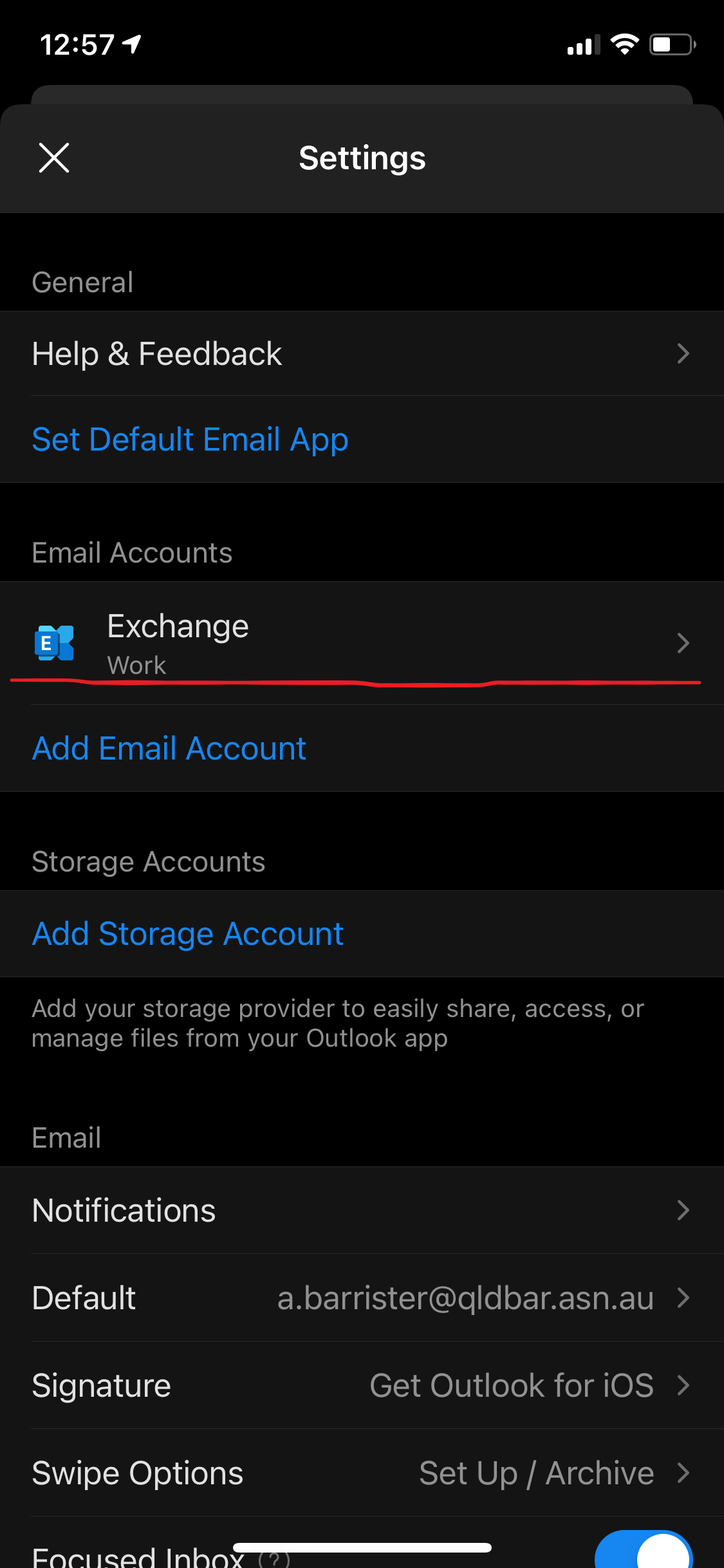This is a detailed caption of a cell phone screenshot:

"The screenshot captures a cell phone’s settings menu displayed at 12:57 PM, as indicated by the clock icon on the upper left corner. On the upper right corner, icons for cell phone reception, Wi-Fi connectivity, and battery status are visible. Below this top bar is the settings header with an 'X' icon for closing the menu on the left. Underneath, the header 'General' is prominently displayed, followed by a 'Help and Feedback' option. Subsequently, the option to 'Set Default Email App' is listed.

The next section, 'Email Accounts,' includes an 'Exchange' account labeled 'For Work,' distinguished by a red line added through photo editing. Below this, an option to 'Add Email Account' is present. Following this, the 'Storage Accounts' section offers an option to 'Add Storage Account.' Finally, the 'Email' section provides settings for notifications (currently set to 'Default'), email signature, and swipe options."